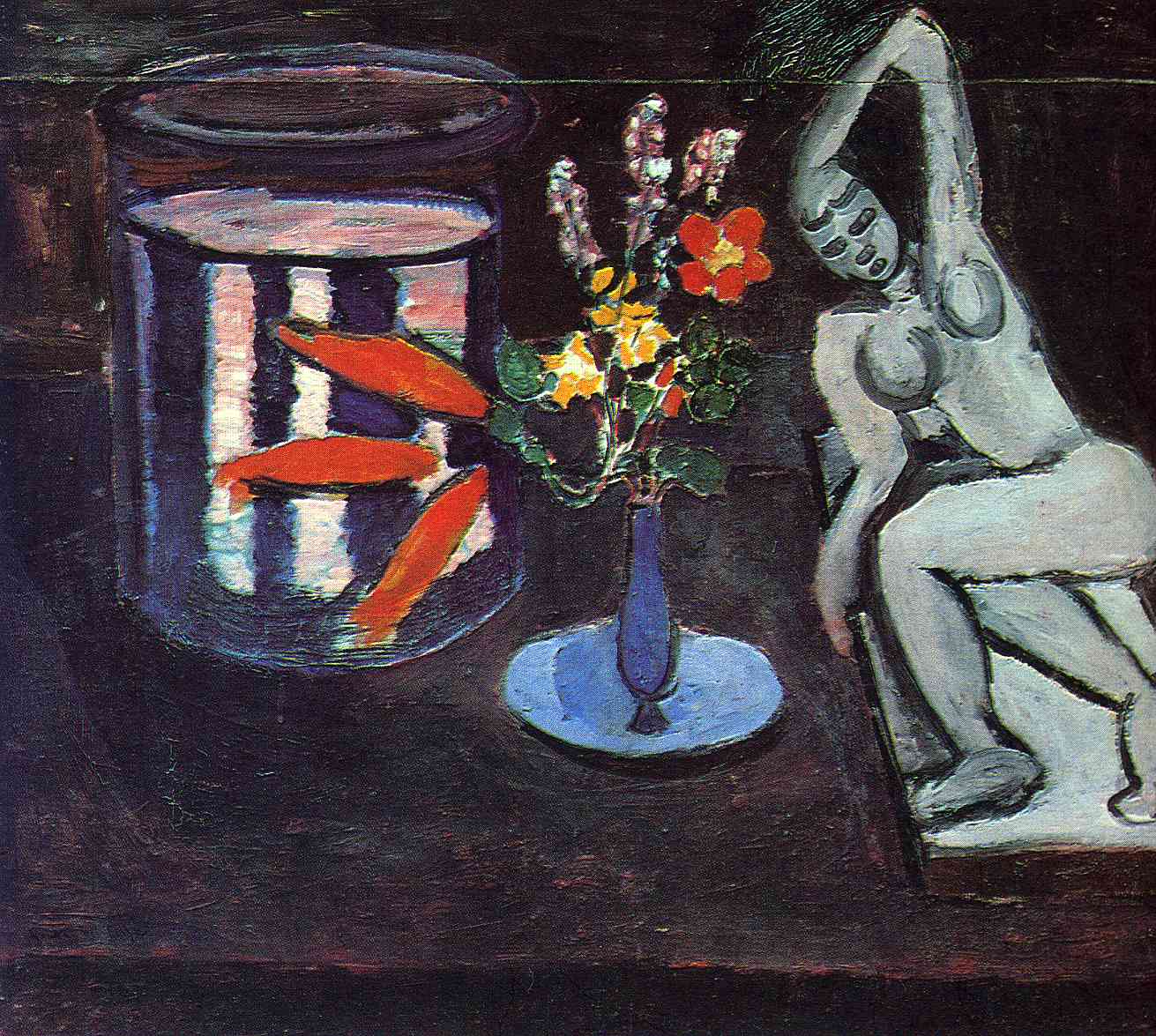The painting features a dark, impressionistic depiction of a tabletop scene set against a background melding shades of blue, gray, and red. On the right side of the table, there's a figurine of a nude woman reclining on her left hip, with her left arm raised to her head, her details softly blurred in a grayish-black hue. In the center of the table, a slender blue vase sits on a light blue plate, holding a vibrant bouquet of flowers: red spikes, yellow-centered blooms, purple and white accents, and pink additions. To the left of the vase is a nearly full glass of water, catching and reflecting the vibrant colors of the flowers. The painting's impressionistic style weaves all elements into a cohesive, dreamlike composition.